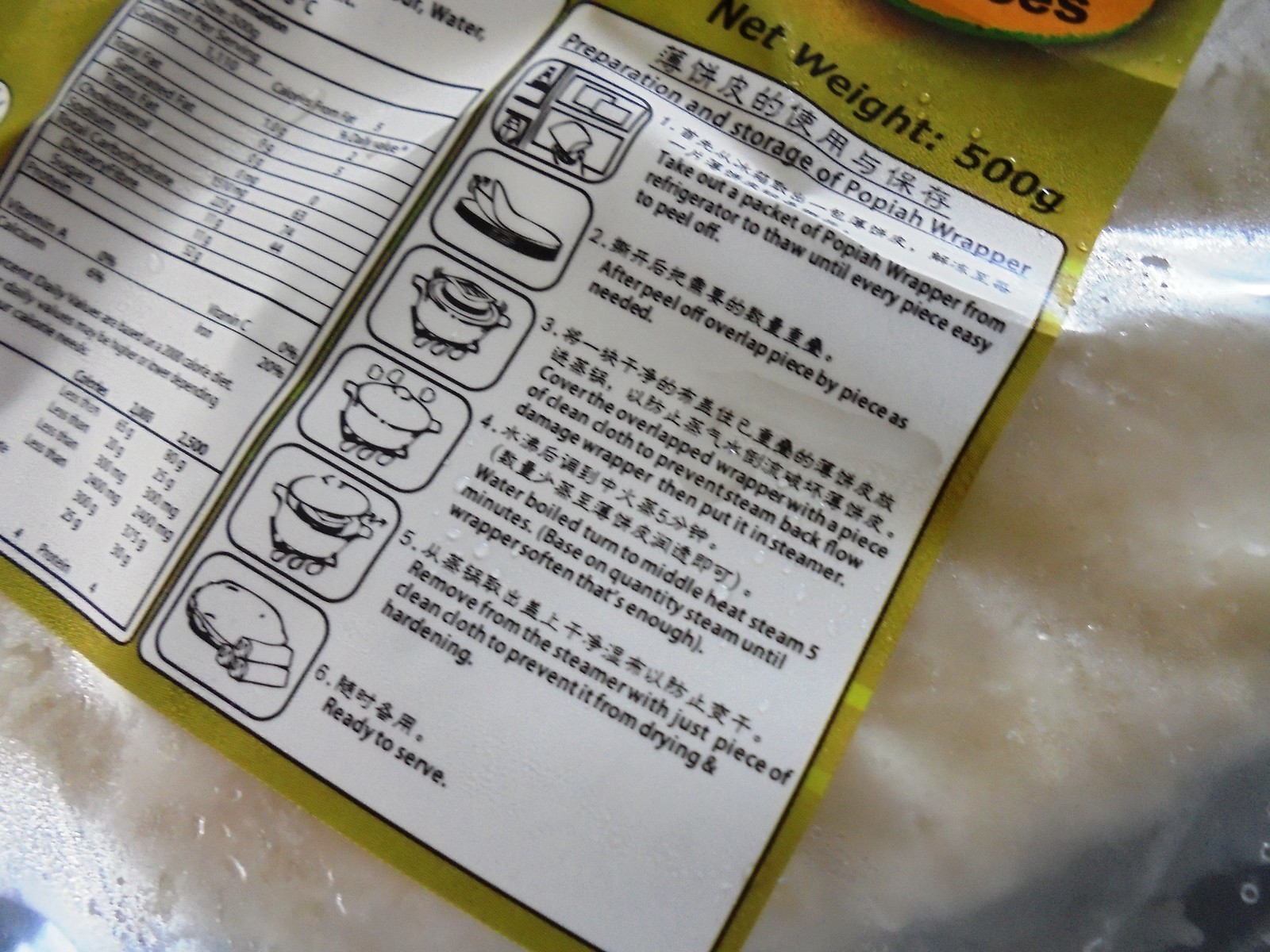This image depicts the back side of a transparent food package, likely Papaya wrappers, taken indoors during daytime. The package has an olive label with white columns and prominently displays "Net Weight 500g" at the top right corner, alongside Chinese characters. The label features a section detailing nutritional facts such as sodium, fats, and vitamin C, though most of the text is in Chinese or Japanese and partially unreadable. A calorie count chart is also visible at the bottom left.

On the right side of the label, there are six illustrated preparation steps with accompanying English instructions. These steps explain how to prepare the wrappers: starting with thawing the packaged wrappers, overlapping each piece, covering with a cloth to prevent steam backflow, steaming for five minutes once the water boils, and finally, removing from the steamer with a cloth to prevent drying. The detailed illustrations include depictions of hands, a pot on a portable stove, and steamer setup, culminating in a final image showing the ready-to-serve wrappers.

Overall, the package appears to contain white-colored food items that are difficult to identify precisely, but the detailed instructions suggest a thoughtful and thorough process for preparing this culinary item.